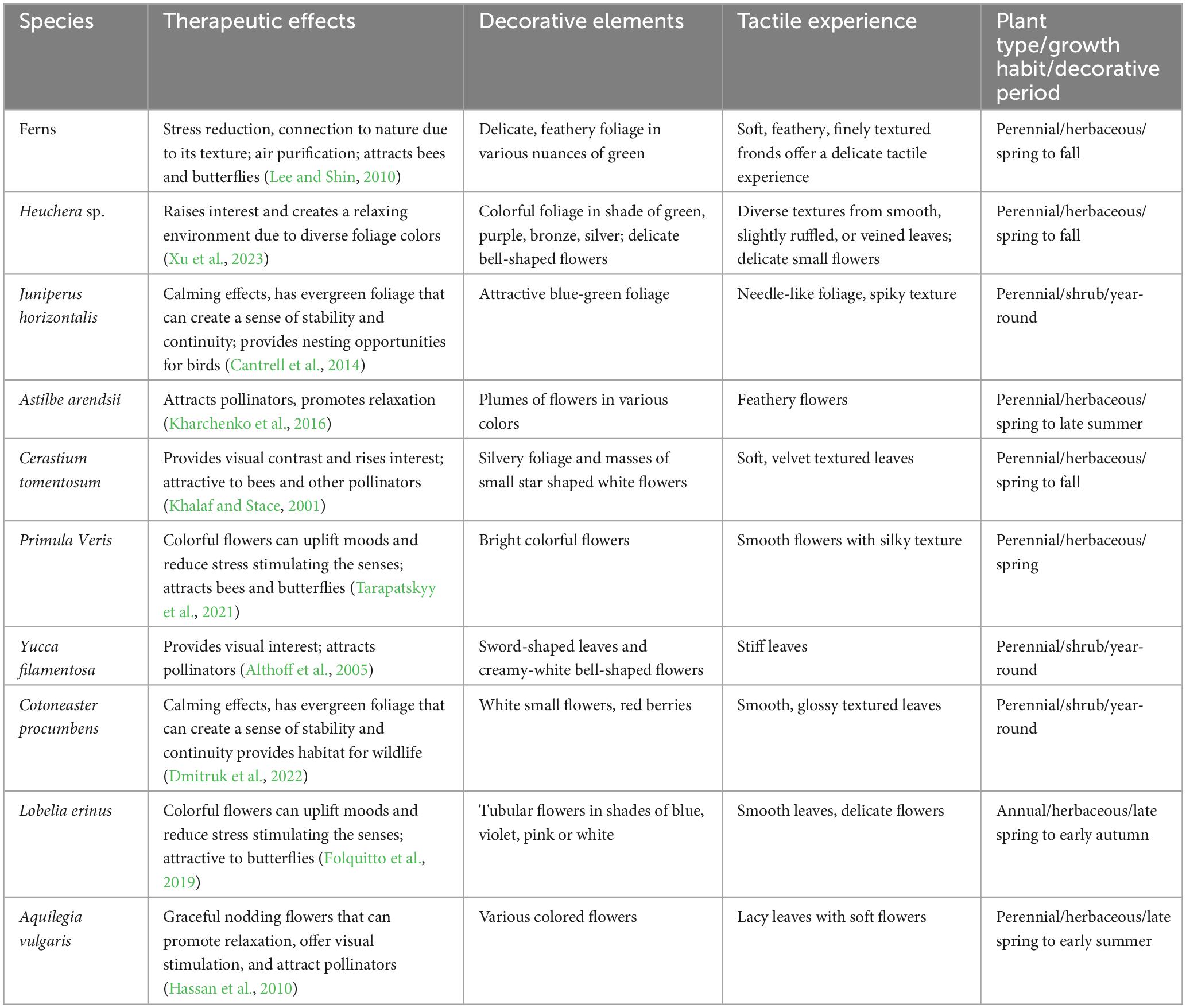The image is a detailed, black-and-white informational chart designed to outline various plants and their characteristics. The chart's header bar is gray with white text and consists of five columns labeled "Species," "Therapeutic Effects," "Decorative Elements," "Tactile Experience," and "Plant Type/Growth Habit/Decorative Period." The leftmost column, under "Species," indicates different plants, including ferns, junipers, yucca, and others, along with their scientific names like Juniperus Horizontalis and Astilba Aranduce. Each row provides specific information for each plant species across the different columns. For example, ferns are noted for their stress-reducing therapeutic effects, delicate feathery foliage for decoration, and a soft, feathery tactile experience. The chart is laid out similarly to a blown-up Excel sheet, with the gray header and white boxes below, each filled with corresponding details about the plants. The layout is simplistic yet comprehensive, making it easy to reference each plant's uses and characteristics.